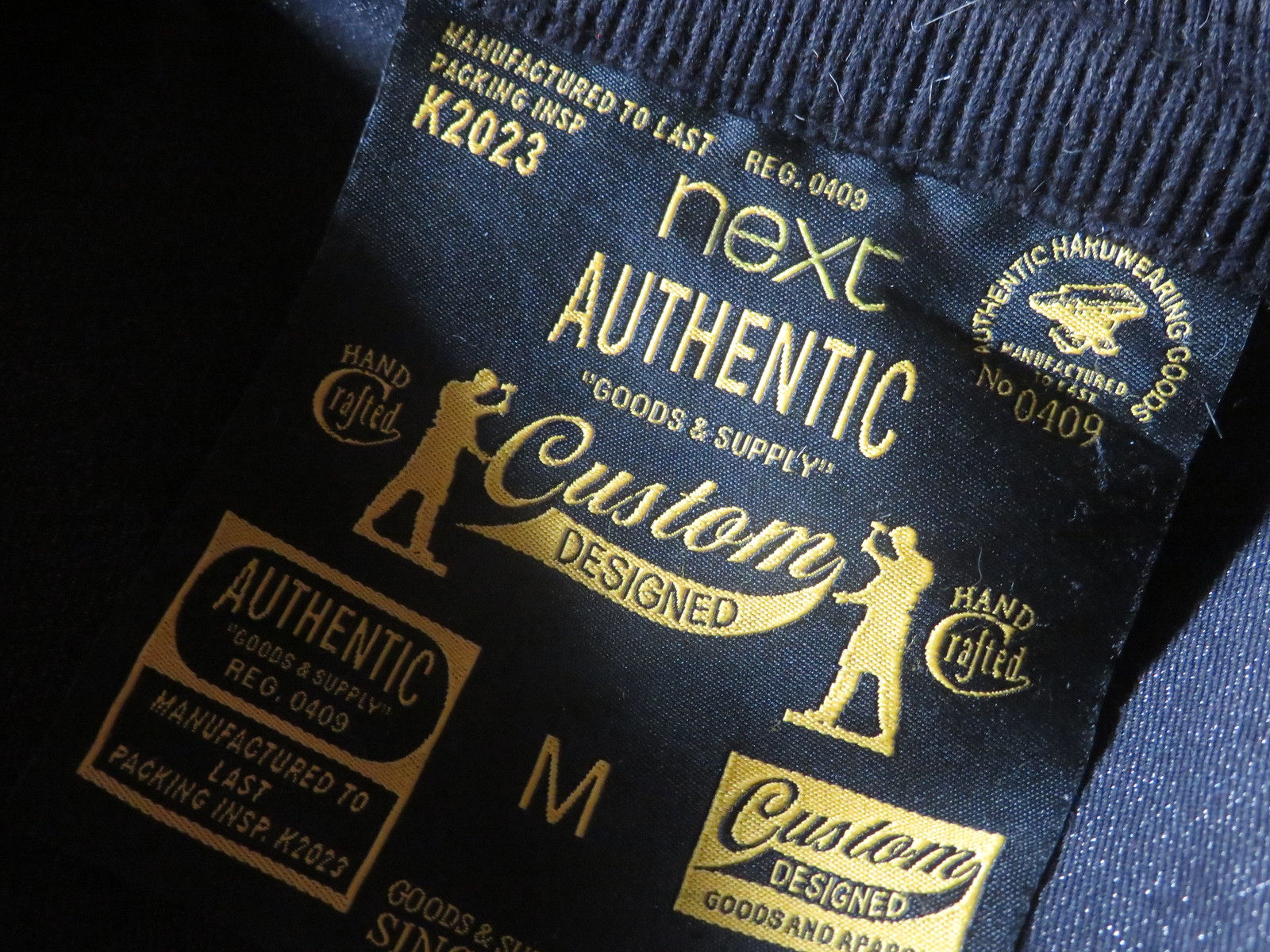The image features a detailed, close-up view of a clothing tag attached to the collar of a dark blue t-shirt. The tag itself is a dark blue or black background with gold-colored text and logos. The central part of the tag displays the text "Manufactured to Last," "Packing INSP K2023," and "RAG0409." Below this, it reads "Custom Designed" with "Next Authentic Goods & Supplies." The design includes an illustration of two figures with hammers on either side of the "Custom Designed" text, giving it a noble, handcrafted appearance. A large "M" is prominently displayed, indicating the shirt size as medium. Additional details include "Authentic Haru-Wearing Goods" and an anvil logo, emphasizing the theme of durability and craftsmanship. The tag is photographed slightly diagonally with a bit of light shining on it, enhancing the textured look of both the tag and the shirt fabric.